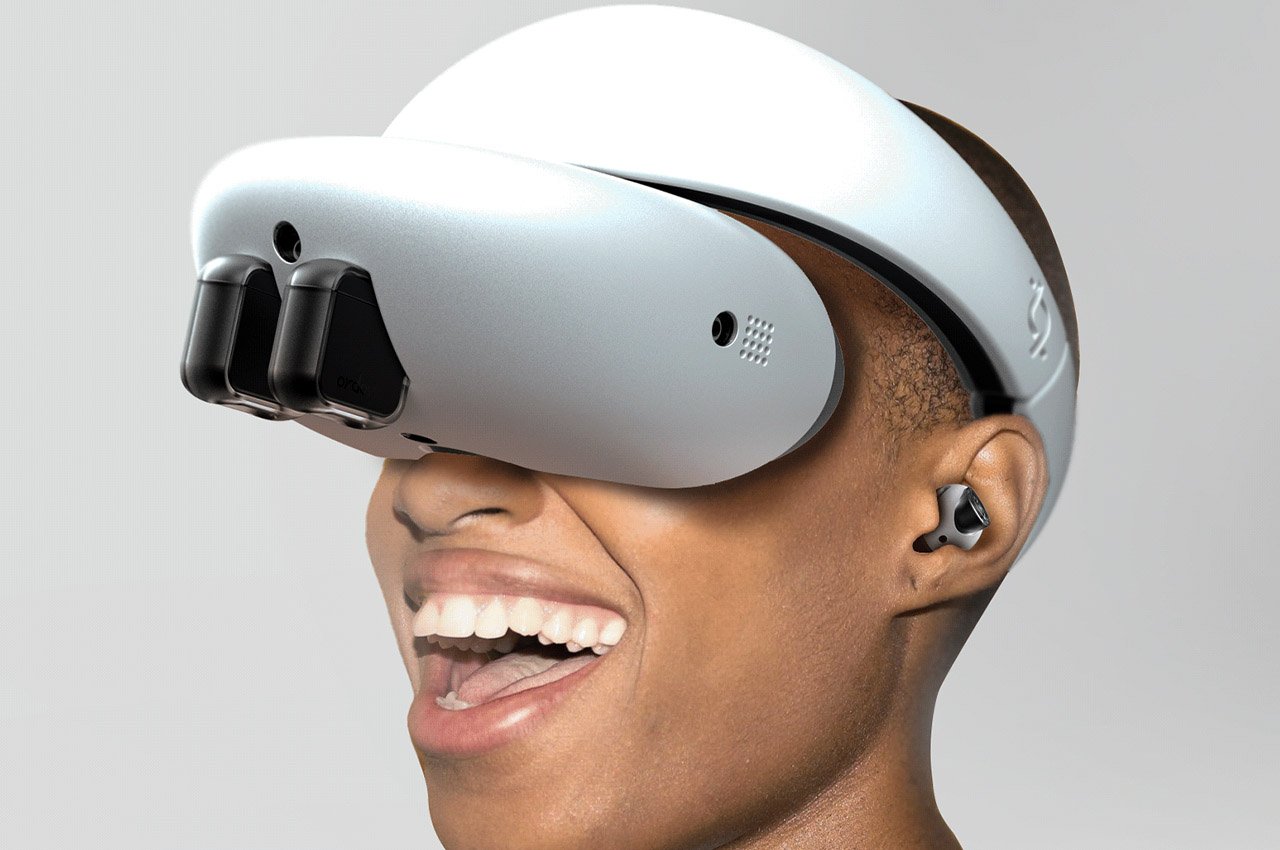This image showcases a dark-skinned person, likely a woman, with a closely shaved or nearly bald head, enjoying an immersive experience with a VR headset. The large, white, rounded VR headset, featuring two black pieces extending from the front, obscures the person's eyes but allows a view of her open mouth, smiling broadly with perfect teeth. A faint logo with intersecting loops is visible on the side of the headset, though it's not clearly identifiable. She also wears a gray and black wireless earpiece. The person is captured in an almost profile view, facing the left side of the image. The background is a faded gray, and the image is well-lit, resembling a professional stock photo. The visible delight on her face suggests she is thoroughly enjoying whatever she is experiencing in this virtual reality environment.